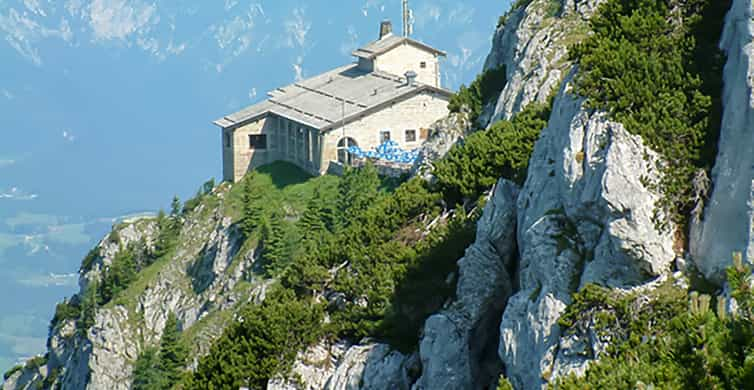Perched on a craggy mountainside, the image captures a one-story building made of pale tan brick with a white sloped roof. The structure, which might be a large house or possibly a church, features an arched window with a cross and several square windows. Toward the back right, a small tower with a chimney and a spire adds to the unique architectural design. The building stands out on a rocky outcrop with a sheer cliff in front of it, dropping off sharply to the left. In the foreground, multiple trees and patches of greenery are visible, complementing the gray rocky cliff face. Blue umbrellas can be seen toward the front of the structure, adding a splash of color. The backdrop reveals a deep, hazy valley with jagged, bush-covered mountains extending toward the right above the building, creating a dramatic and picturesque scene.